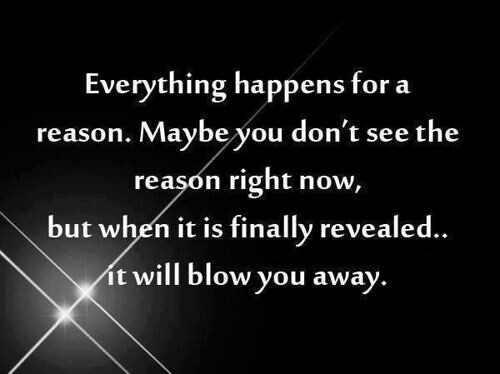The image is a minimalist, black-background digital creation featuring a motivational quote in white lettering at its center. The quote reads, "Everything happens for a reason. Maybe you don't see the reason right now, but when it is finally revealed, it will blow you away." In the lower left-hand corner, there are two intersecting lines of light, resembling a brilliant, star-like gleam or headlights creating an X or cross pattern. These beams start mid-way on the left side and extend diagonally downward, mimicking the look of twinkling lights against the dark backdrop. The white text stands out boldly, providing a stark contrast to the deep black background, making the entire composition visually striking and thought-provoking. This poignant, straightforward design lends itself well to being a motivational quote often seen on social media.